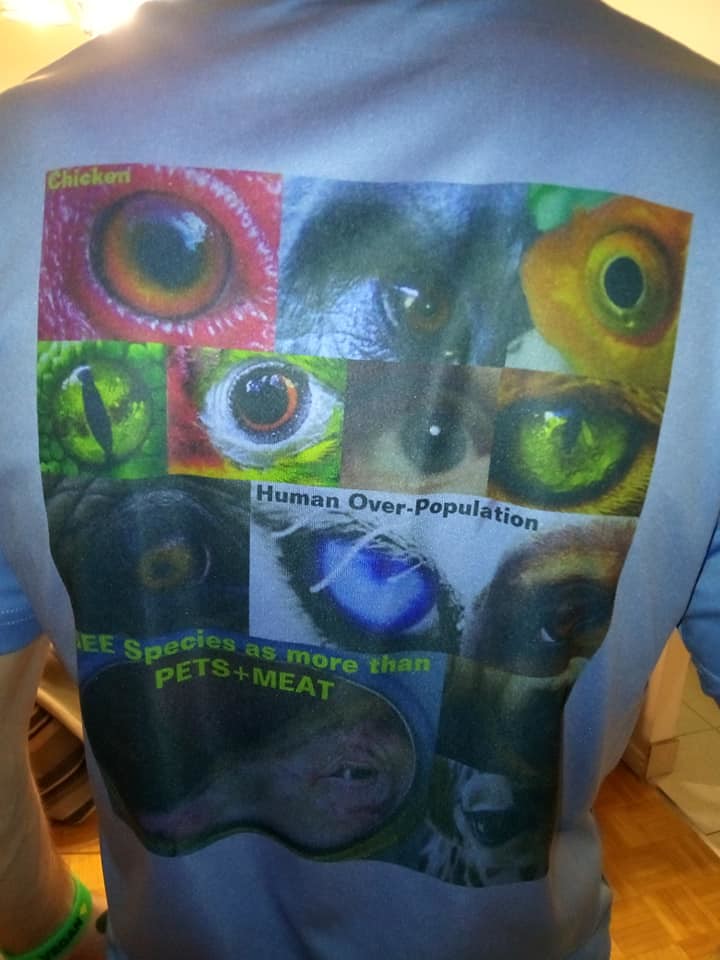The photograph, taken indoors, captures a man standing on parquet wood floors near a doorway framed in white molding. In the right corner of the image, tiles are visible. The man, facing away from the camera, wears a short-sleeved light blue T-shirt adorned with a vibrant array of images on the back. His left arm, partially visible, is relaxed at his side and adorned with a green wristband, while his right arm is out of sight. The T-shirt's back displays a colorful collage of animal eyes, starting with a chicken's eye in the upper left corner, followed by a green fish eye and a goldfish eye. The second row shows four different animal eyes, the third row features three, and at the bottom of the shirt, a tiger's head with a pair of goggles is displayed. Below the tiger's head, the shirt carries a message: "see species as more than pets and meat."